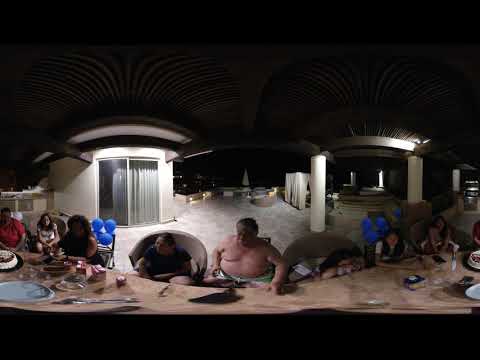The image captures a nighttime celebratory event, likely a birthday party, set outdoors under a dark sky. A long brown table stretches across the lower half of the scene, adorned with plates, utensils, and cakes. The central figure, a heavyset older man dressed only in beach shorts, sits shirtless at the table. To his left sits an older woman, with more people — including four adult women and some young ladies — arranged on either side of the table, all engaged in the festivities. Blue balloons are attached to the back of one of the chairs, adding to the festive atmosphere. In the background, white pillars and a white building with an illuminated sliding glass door, possibly a pool area, suggest the location, with umbrellas and minimal lighting from the surrounding structures.